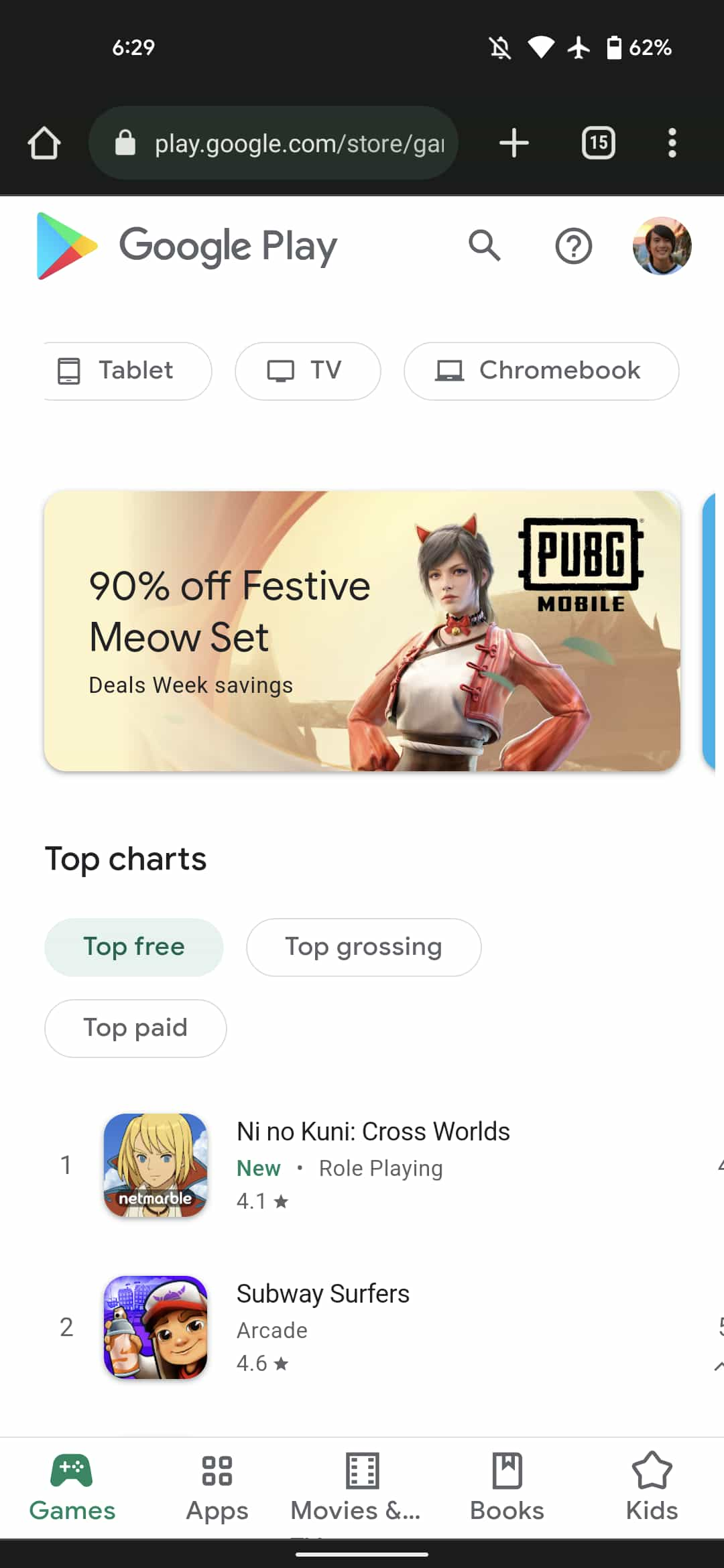A close-up image of a smartphone screen displaying the Google Play Store is shown. The device is in airplane mode with a 62% battery level and is connected to Wi-Fi. The URL at the top of the screen reads "play.google.com/store/gay...", which is incomplete. The screen features a predominantly white background with the words "Google Play" written in black at the top center.

Below the "Google Play" heading, there are various interactive buttons, including "Search", a "Profile picture", "Tablet", "TV", and "Chromebook". An advertisement banner is visible, promoting a "90% off Festive Meow Set, Deal Week Savings" for PUBG Mobile.

Further down, the interface shows navigation options: "Top Charts", "Free Top", "Top Grossing", and "Top Paid". The "Free Top" section is highlighted in green, and the first app listed is "Ni no Kuni: Cross Worlds", marked as new, categorized under Role Playing with a 4.1-star rating. The second app listed is “Subway Surfers”, categorized under Arcade with a 4.6-star rating.

At the bottom of the screen is a navigation bar with options: "Games" (highlighted in green), "Apps", "Movies & Books", and "Kids" (all grayed out). The bottom edge of the screen features a distinct black line completing the interface.